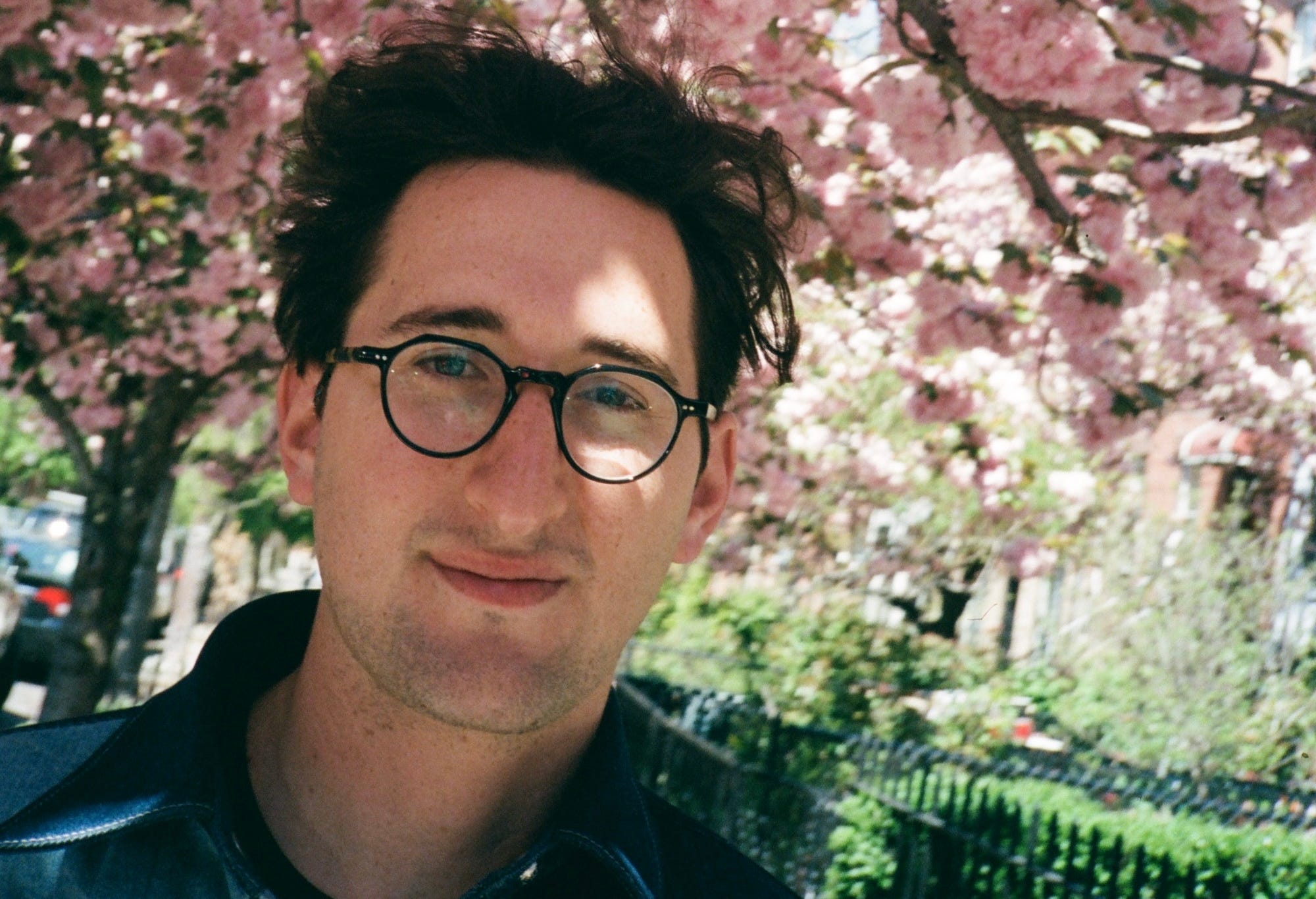This close-up, rectangular photograph captures a man in his late 20s to early 30s, who occupies much of the frame, leaning slightly in from the left. He has long, swept-back dark hair and small, round black-rimmed glasses, accentuating his dark blue eyes. His face, featuring a faint stubble on his chin and a very slight smile, is distinctly Caucasian. He is dressed in a dark blue shirt, possibly layered with a black jacket, visible just below his neck. The background, though blurred to keep the man in sharp focus, reveals a beautifully lit spring scene. Pink dogwood trees in full bloom dominate the top third of the image, spreading across the width with their vibrant blossoms. Beneath them, greenery and low-lying bushes blend with a low, black iron fence. To the man's left and slightly behind the tree, a parked car is faintly visible, hinting at a picturesque park or street scene basking in sunlight.